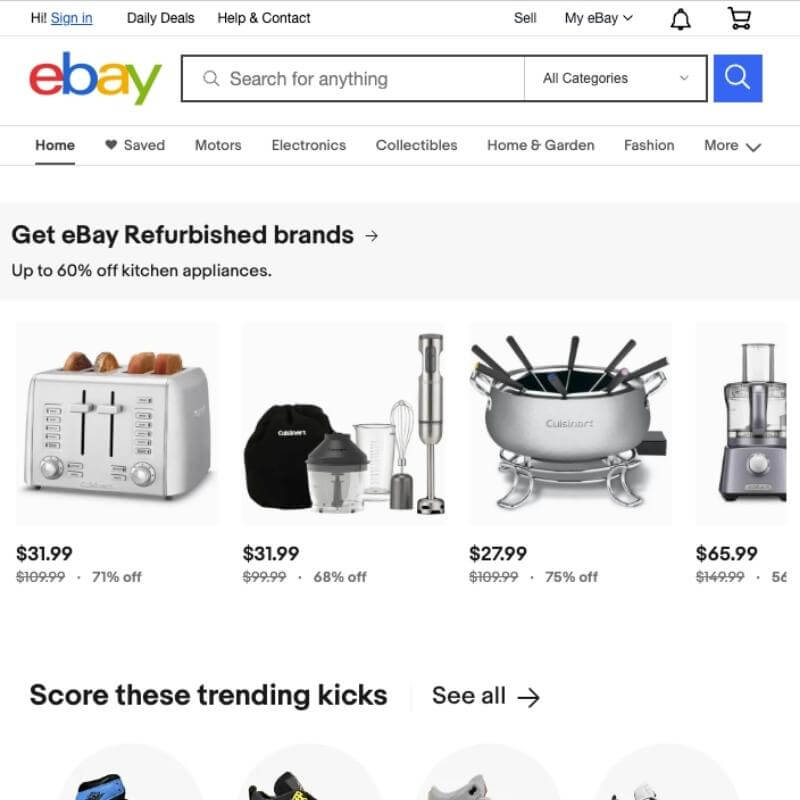In the provided image, there is a screenshot of an eBay webpage. At the top of the page, there is a black navigation bar. On the top left, there is a hyperlinked "eBay" logo followed by options such as "Daily Deals," "Help & Contact," all separated by the ampersand symbol. Further to the right, you find options labeled "Sell" and "My eBay," accompanied by a drop-down arrow. Toward the far right side, there are notification and cart icons.

This header area is bordered on the bottom by a thin, continuous red line. Adjacent on the left is the eBay logo in lowercase letters: ‘e’ in red, ‘b’ in blue, ‘a’ in yellow, and ‘y’ in green. Moving to the right, there is an empty search bar which displays placeholder text, “Search for anything,” in light gray, alongside a small magnifying glass icon. A vertical break separates this from a drop-down menu reading “All Categories” next to a light blue square containing another white magnifying glass icon. 

Directly beneath this, there is a secondary navigation bar in light gray featuring links to various categories: "Home" (highlighted in black), "Saved," "Motors," "Electronics," "Collectibles," "Home & Garden," "Fashion," and more. A promotional overlay below this section announces “Get eBay Refurbished Brands” in bold black text followed by a right arrow, with a subtitle offering “up to 60% off kitchen appliances.”

The main section shows images and details of discounted kitchen items. On the left is a picture of a toaster priced at $31.99 in bold text, reduced from $109.99 (71% off). To its right is a kitchen set originally priced at $31.99, now $9.99 (68% off). Continuing to the right is a fondue set priced at $27.99, reduced from $109.99 (75% off). Lastly, there is a juicer listed at an indistinguishable price, previously marked at $149, with the remaining price cut off from view.